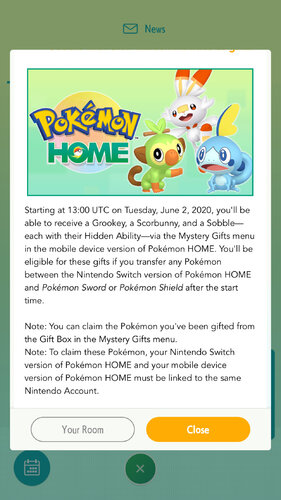A screenshot of the Pokémon Home website captured on a mobile device. The background features a gradient transitioning from a dull puke green at the top to a light teal green towards the bottom. At the top of the page, a small green letter is displayed next to the word "News," both in green text. The header announces the availability of new Pokémon with hidden abilities, starting from 13:00 UTC on Tuesday, June 2, 2020.

The main section of the page showcases Pokémon Home with several different Pokémon pictured inside—specifically a green monkey (Grookey), a white rabbit (Scorbunny), and a blue lizard (Sobble). The Pokémon logos are prominently displayed in yellow and blue colors. Situated in the center of the Pokémon Home is a miniature Pokéball.

The accompanying text details that users will be able to receive Grookey, Scorbunny, or Sobble with hidden abilities via the Mystery Gifts menu in the mobile version of Pokémon Home. To be eligible for these gifts, players must transfer their Pokémon between the Nintendo Switch version of Pokémon Home and Pokémon Sword or Pokémon Shield at the designated start time. The gifted Pokémon can be claimed from the Gift Box in the Mystery Gifts menu. It is important to note that both the Nintendo Switch version and mobile device version of Pokémon Home must be linked to the same Nintendo Account.

Additional navigation buttons are present on the page, including a circular button for your room, an orange button with white text that says "Close," a calendar button on the bottom right-hand side, and a dark green "X" button at the bottom of the page.